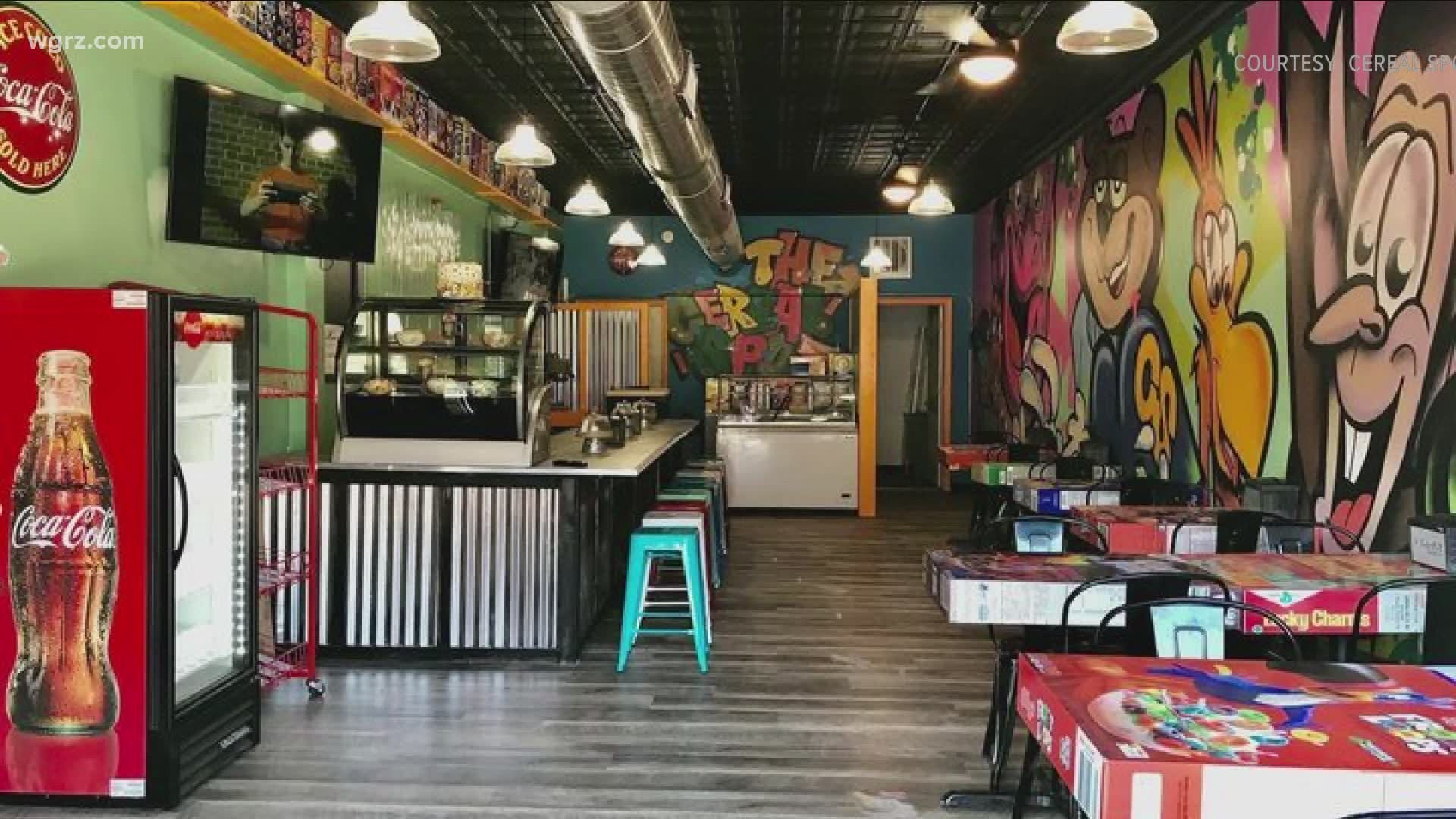The photograph depicts the interior of a small, nostalgic-themed restaurant that exudes the charm of an old-time coffee shop. Prominently, a counter area stretches across the center of the image, equipped with several crude bar stools without backs, offering seating for five or six people. Above the counter, there is a bakery shelf that displays a selection of pastries within a glass container. To the left of this counter sits a Coca-Cola vending machine, accompanied by an overhead Coke advertisement, and a television mounted on the wall.

Dominating the right side of the image, there's a whimsical mural featuring various cartoon characters like Count Chocula and Toucan Sam, adding an element of fun and nostalgia. The series of four-top tables lined against this muraled wall are uniquely designed to resemble giant cereal boxes, including popular brands like Froot Loops, Lucky Charms, and Cocoa Puffs. The tables are surrounded by black chairs, contributing to the eclectic atmosphere. Additionally, dome-shaped white lighting fixtures hang from the ceiling, illuminating the whole dining area.